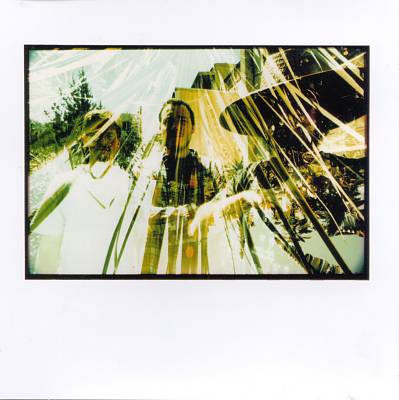This is an abstract, somewhat distorted photograph that could be an album cover. It features three men standing in front of a cityscape with trees and buildings in the background. The photograph is characterized by strong sunbeams that pierce through, obscuring much of the detail and making it difficult to discern the faces clearly. The image is framed in black.

The man on the top right wears a straw hat, sunglasses, a black shirt, and sports a brown beard. The central figure, with a receding hairline, has short black hair and a beard around his chin, and is dressed in a plaid long-sleeve shirt. The man on the left, with medium brown hair, is clad in a white t-shirt. There's a mix of green, yellow, tan, white, and light blue colors in the palette, adding to the sunset or sunrise effect meant to evoke a spiritual or artistic ambiance. Despite the vibrant colors and artistic attempt, the heavy beams of light detract from the clarity of the overall image. This photograph lacks any identifying information, such as dates or names.